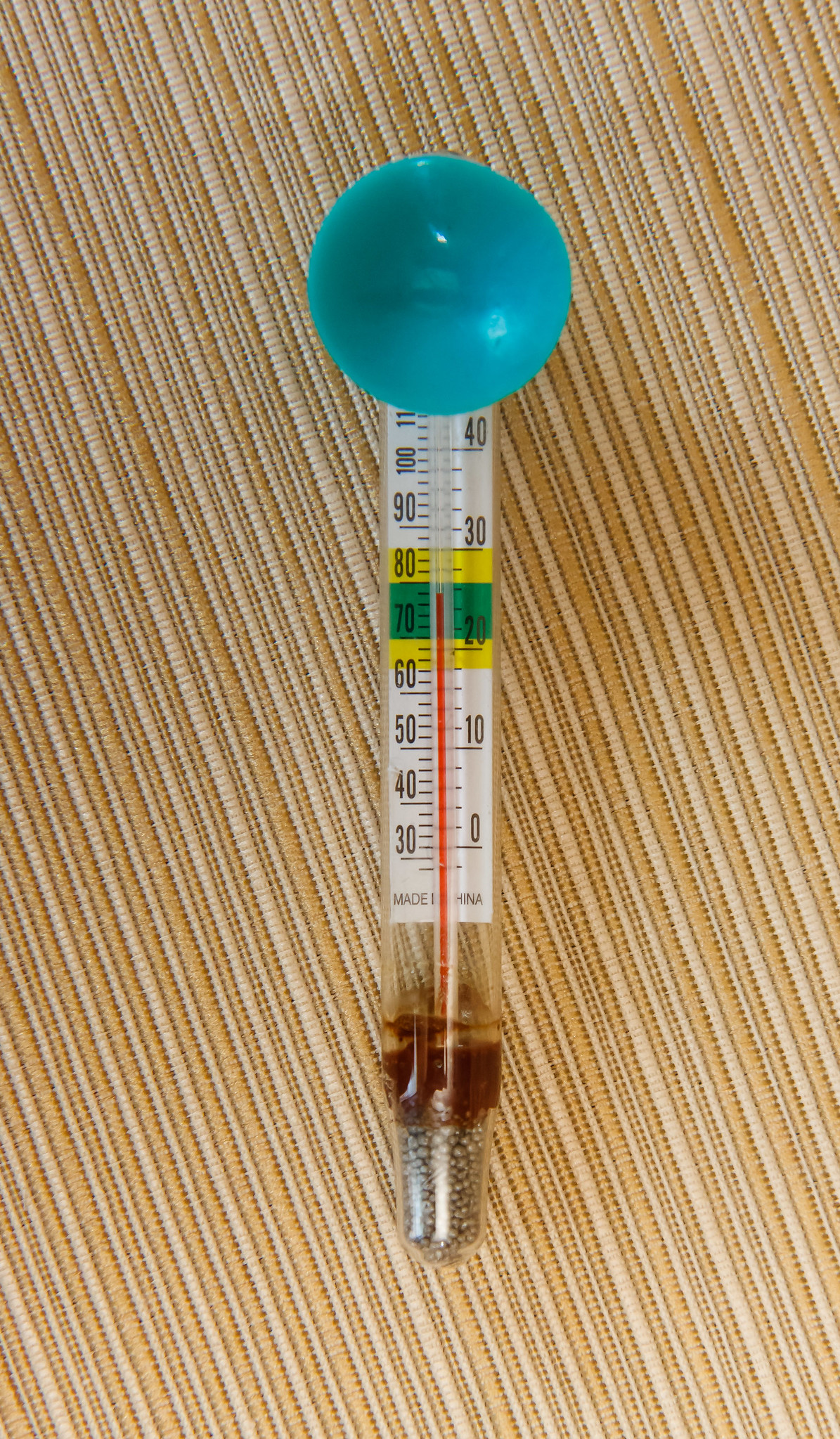This is a detailed photograph of a rectangular, portrait-oriented glass thermometer. The thermometer, designed for indoor or culinary use rather than outdoor temperature measurement, has a sleek silver tip at the bottom and a turquoise ball at the top, which serves as a decorative and functional end cap. The instrument is vertically oriented, with a clear glass tube displaying temperature readings.

The left side of the thermometer is marked with numbers that start at 30 degrees at the bottom and ascend incrementally up to 110 degrees, although the highest digits are partially obscured by the turquoise ball. This side likely represents Fahrenheit degrees. On the right side, the thermometer shows a scale marked from 0, increasing in increments of 10 up to 40, which suggests it is indicating Celsius degrees.

In the center of the thermometer, there is a distinct color-coded section. A green zone, surrounded by two yellow sections, spans approximately from the mid-60s to the mid-80s Fahrenheit. This likely indicates an optimal temperature range for a specific purpose, such as cooking or candy making. The green section is notably broader than the flanking yellow sections, emphasizing its significance as a target zone.

The thermometer bears a "Made in China" label, adding a note of provenance to its detailed and functional design.